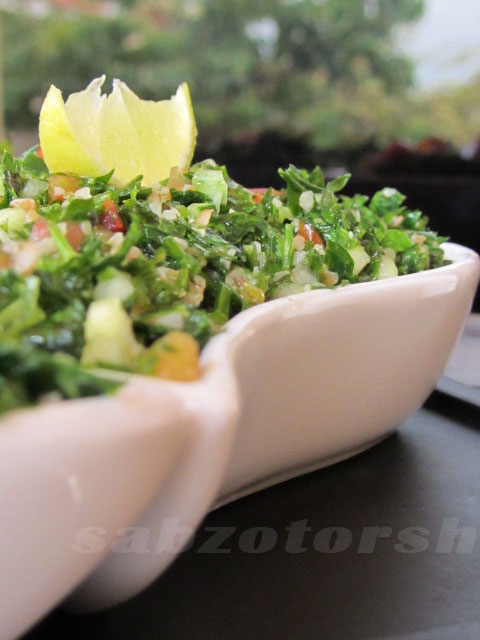This image is a detailed close-up of a dish named Sabzotorsh, presented in a white, uniquely shaped ceramic bowl. The dish appears to be a finely chopped salad or condiment, featuring a blend of various colors and textures. Key ingredients are evident through the vibrant greens, along with red, white, and orange specks, all meticulously mashed together. An upright lemon wedge is prominently placed on top, adding a fresh, zesty accent to the dish. The background, blurred to keep the focus on the food, suggests an outdoor setting with sunlight filtering through trees, leaves, and plants, hinting at a natural and inviting environment. A black table sign and a watermark with the name "S-A-B-Z-O-T-O-R-S-H" are also noticeable in the image, providing further context and authenticity.